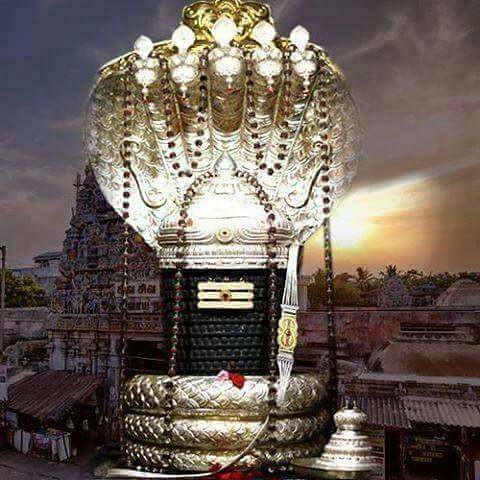The photograph captures a striking scene featuring a metal or metallic decorative Asian building adorned with intricate designs that resemble beads. Striking lights highlight this prominent structure, making it stand out against the surrounding darkness and shadow-enhanced scenery. To the left, another ornate, square-shaped building embellished with jewel-like beads also reflects traditional Asian design elements. 

The centerpiece of the image is a majestic black statue of the Hindu deity Shiva, crowned by a five-headed snake coiled in layers of gold and silver. This divine figure is marked with three white stripes and a red dot on its forehead, and is surrounded by red and pink flowers. A cityscape unfolds in the background, with a temple visible on the left and a cluster of shops at the bottom left. The sky in the distance is alive with the hues of a sunrise, from brilliant blues and oranges to radiant yellows, lending a celestial glow to the entire scene.